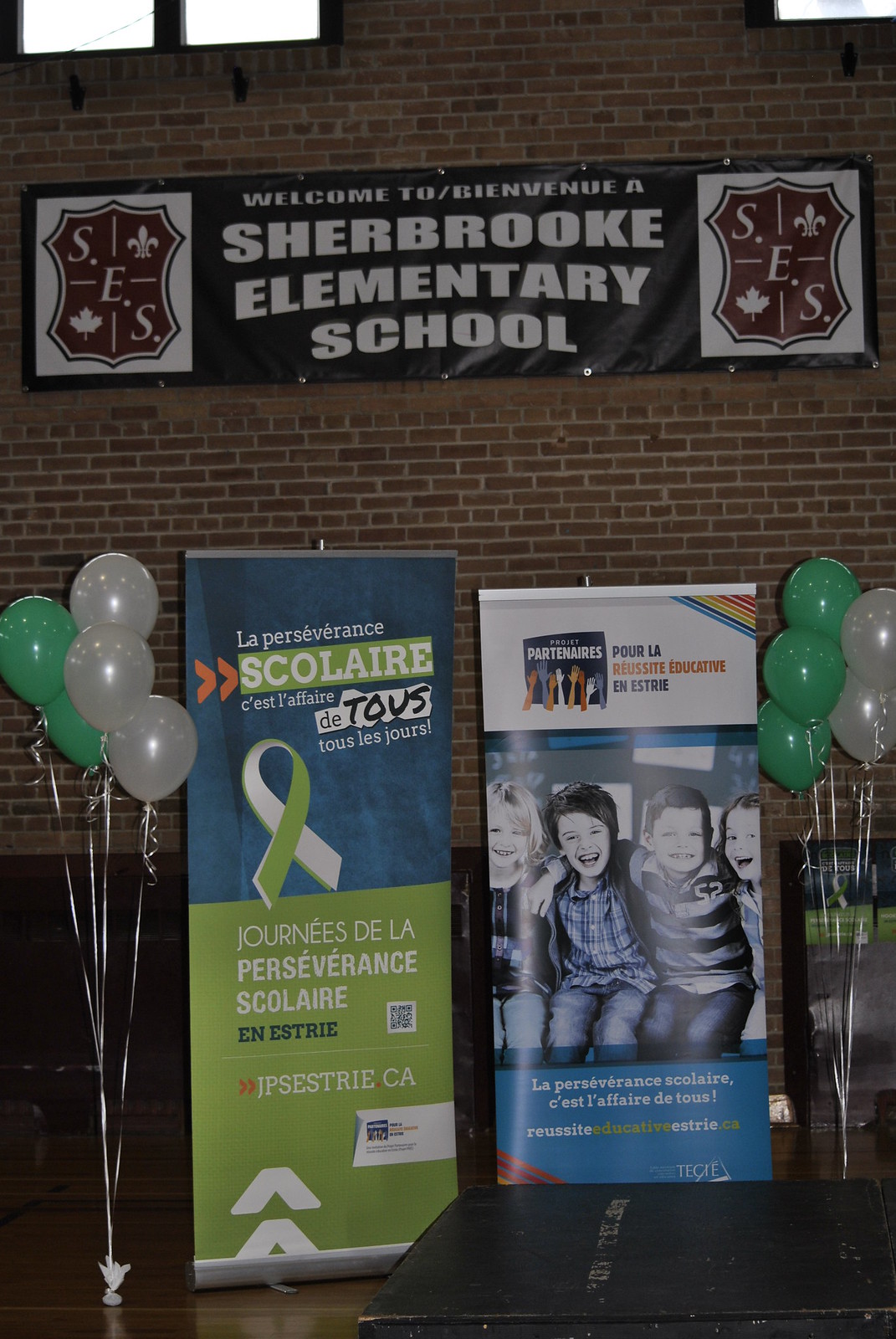The image depicts an indoor scene at Sherbrooke Elementary School, with a red brick wall serving as the backdrop. At the top of the image, three windows let in natural light. Dominating the middle of the scene is a horizontal black banner with white text that reads "Welcome to Bienvenue à Sherbrooke Elementary School." On either side of the banner are logos featuring shields, each with the letters "S.E.S.", a maple leaf in the bottom left corner, and a fleur-de-lis in the top right corner, indicative of its Canadian location.

In front of the brick wall, there is a brown table adorned with banners and flanked by green and white balloons. The left banner is blue and green and reads "La Persévérance Scolaire," with additional French text detailing the importance of perseverance in education. The right banner features an image of several children joyfully holding each other's shoulders, accompanied by similar supportive text in French. The floor in the scene is brown wood, adding warmth to the indoor setting. Overall, the scene is celebratory and welcoming, emphasizing school spirit and the value of perseverance in academic success.